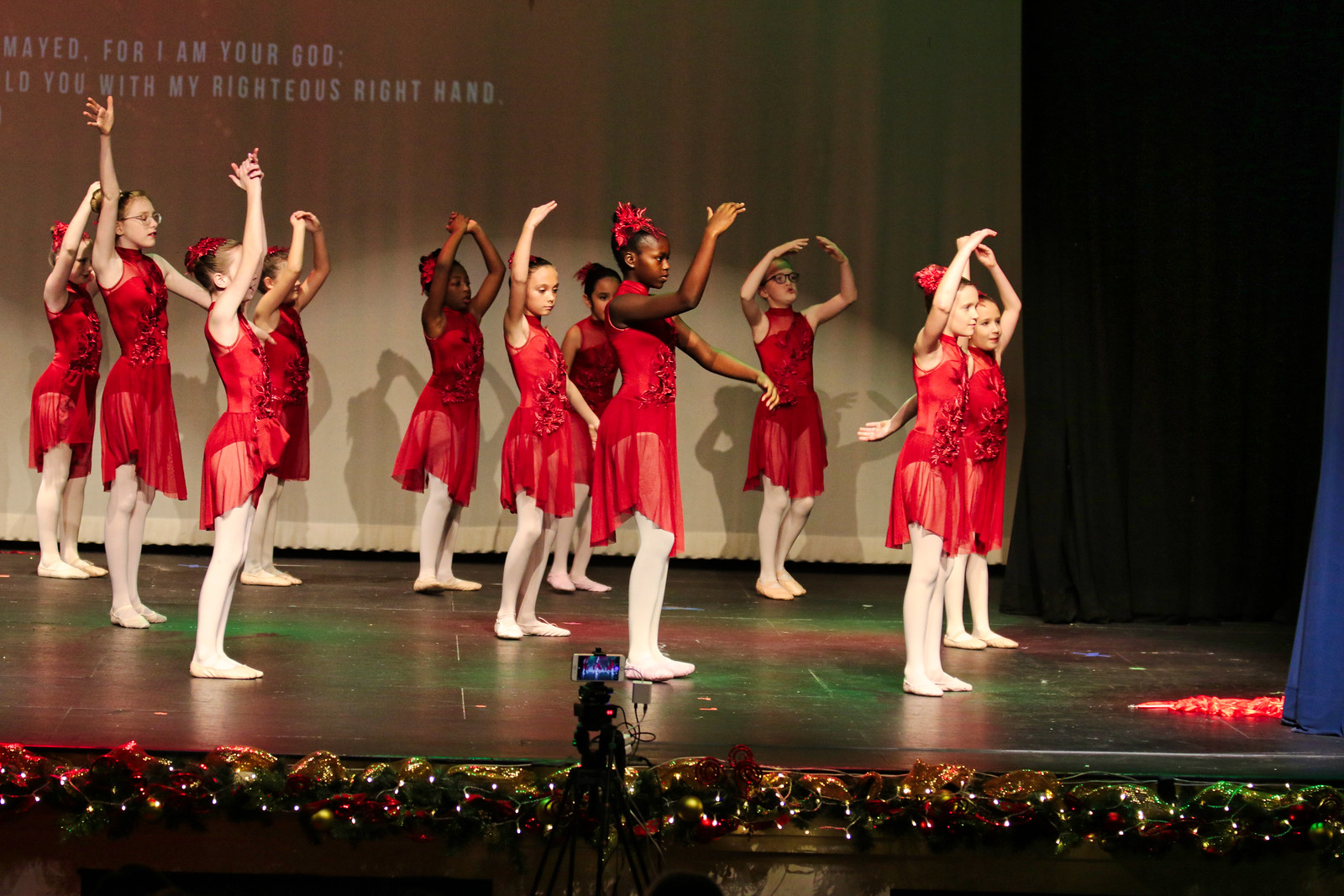The photograph captures a lively indoor stage performance featuring 10 to 12 young girls, approximately 10 years old, dressed in matching sleeveless red leotards with sheer red skirts, white tights, and white shoes. They also have red ribbons adorning their hair. The girls, of primarily Caucasian descent with a few of African descent, appear to be dancing with their arms gracefully raised in a ballerina-like fashion. The stage itself is decorated with a garland intertwined with small decorative lights along the front edge. At the center of the foreground, a tripod-mounted video camera records the performance. Behind the dancers, a large light-colored curtain hangs, partially displaying text that reads, "for I am your God... you with my righteous right hand." The upper right corner behind the stage transitions into a black curtain.